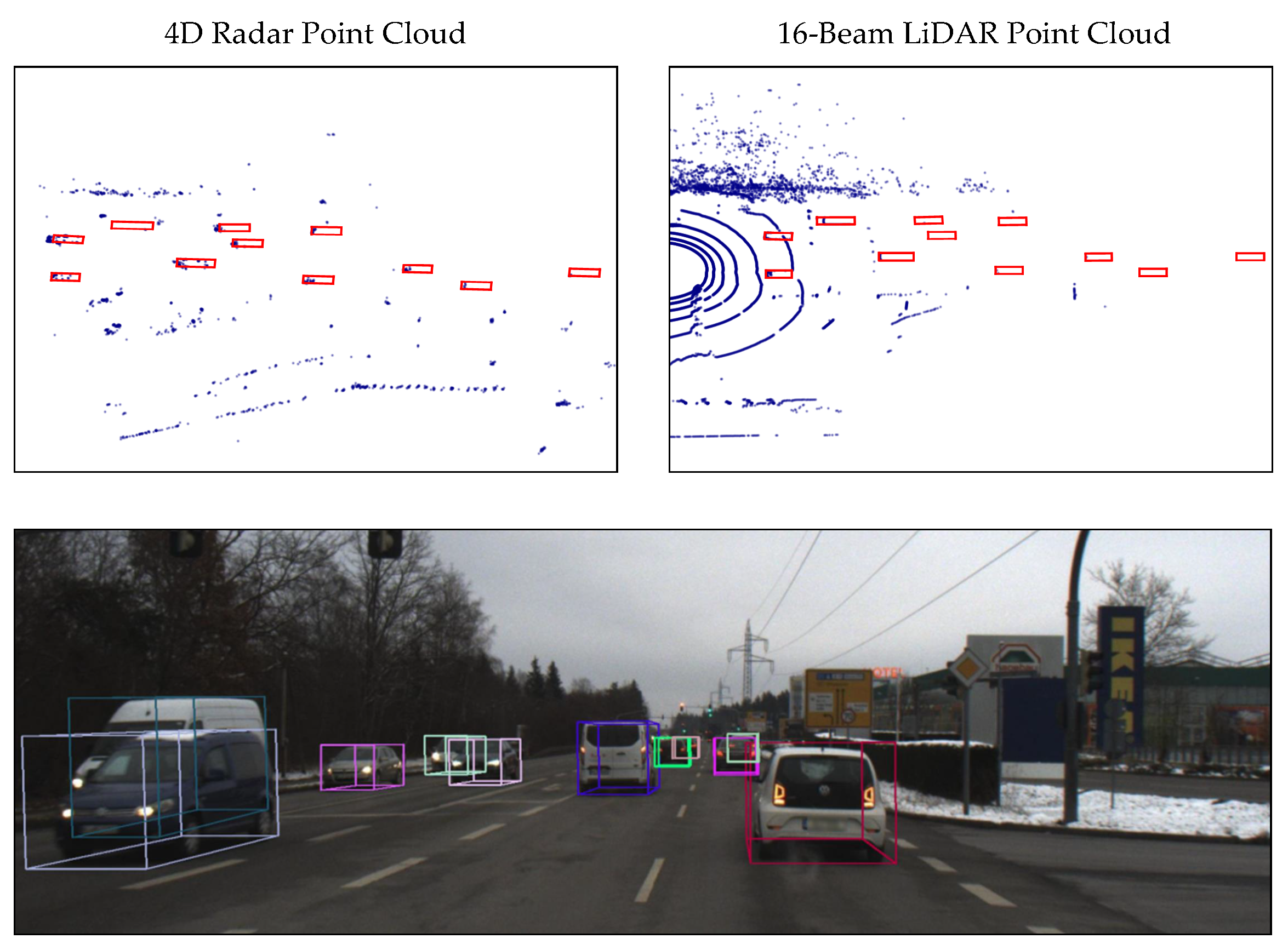The image consists of three sections: two diagrams at the top and a photograph at the bottom. The top left diagram, labeled "4D radar point cloud," features a white background with a black border, and contains small red rectangles interspersed with blue dots and dashes. The top right diagram, labeled "16-beam LiDAR point cloud," also has a white background with a black border, and includes an arrangement of red rectangles with additional features like curved blue lines and blue dots forming a pattern reminiscent of an oval or racetrack.

Below these diagrams is a photograph of a four-lane street, with cars traveling in both directions; those on the right are moving away, while those on the left are coming towards the viewer. Each vehicle is highlighted with different colored bounding boxes—red, blue, green, purple, and gray—signifying their detection by the AI system. The scene also includes an IKEA sign and surrounding buildings on the right side of the road, a tree-lined area on the left, and a median with some snow.